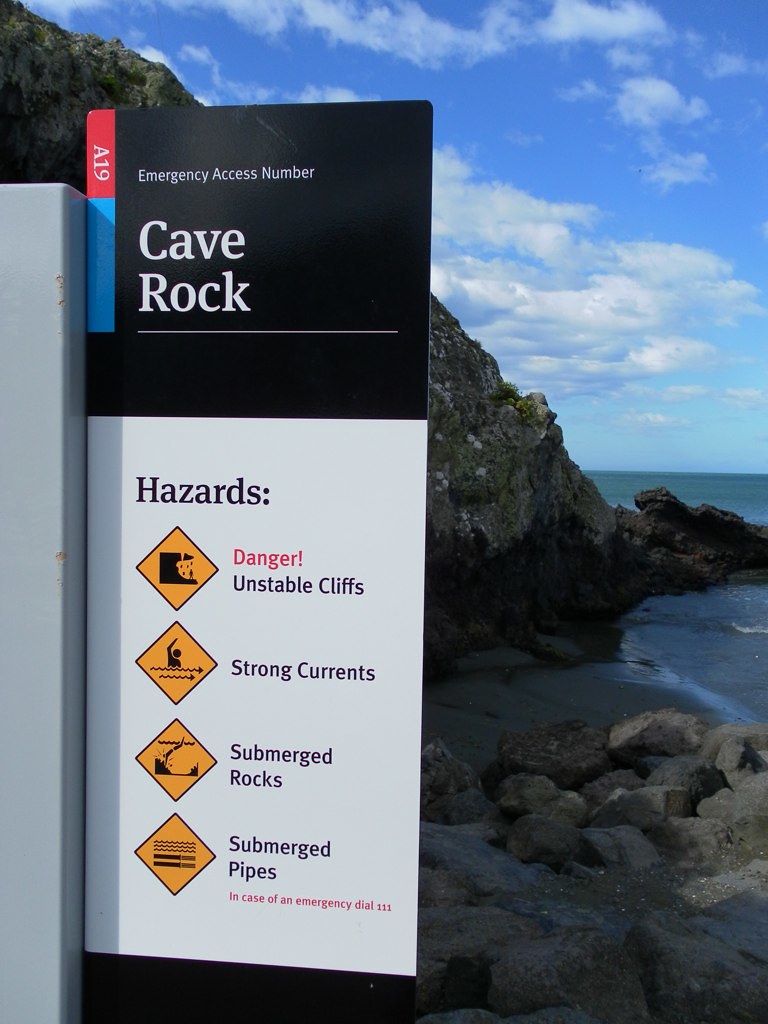In this color photograph, a prominent vertical sign stands on the left side against a stunning seaside backdrop. The top one-third of the sign is black with bold white lettering that reads "EMERGENCY ACCESS NUMBER" above "CAVE ROCK." Adjacent to this, a vertical bar split into red and blue sections prominently displays "A19" in white font on the red portion. The bottom two-thirds of the sign features a white background with the bold heading "HAZARDS," followed by four yellow diamond-shaped warnings stating: "DANGER! UNSTABLE CLIFFS," "STRONG CURRENTS," "SUBMERGED ROCKS," and "SUBMERGED PIPES." The sign is mounted on a vertical gray pole. The scene is set at a rocky beach with large cliffs surrounding the view, a beautiful blue sky filled with puffy white clouds, and water beneath the cliffs. The photographic style is representational realism, capturing the serene yet precarious landscape in vivid detail.